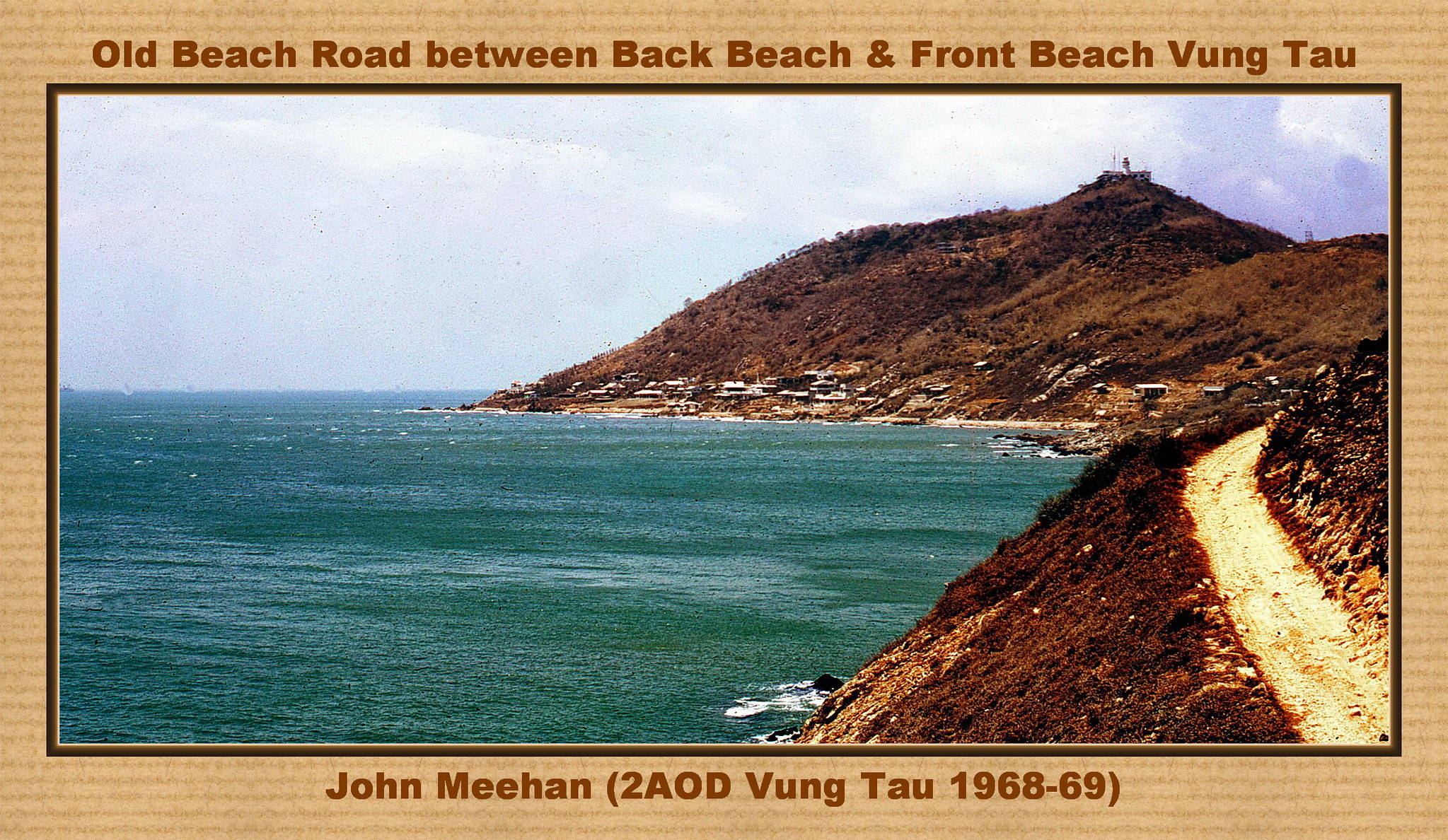This is an old, rectangular-shaped photograph with a dark brown paper border and a cardboard or cardstock texture where fibers of the paper are visible. The top and bottom borders feature text in brown font that reads: "Old Beach Road between Back Beach and Front Beach, Vung Tau." The bottom adds, "John Meehan to AOD Vung Tau, 1968-69." The image captures a seaside view with a calm, blue-green ocean extending from the lower left. On the right, a winding dirt road wraps around a brown-covered hill, likely short grass or weeds. In the distance, small houses or buildings are nestled on the hillside, positioned almost at the shoreline. Overhead, a largely white sky with patches of blue and some clouds hovers above. The waves appear gentle, with slight white caps visible where they meet the shore. This vintage photograph offers a serene glimpse of a tropical landscape, highlighting the tranquil yet rugged beauty of Vung Tau's coast during the late 1960s.